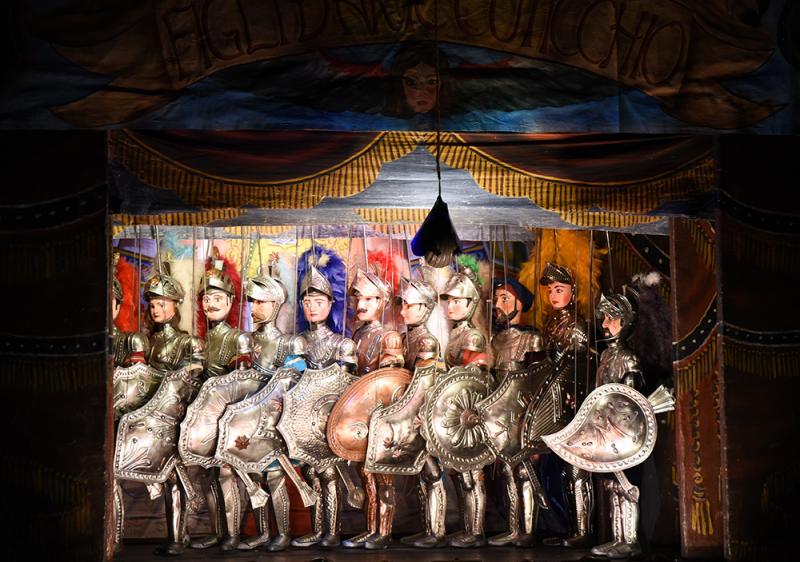In this hand-drawn depiction of a puppet theater play, the forefront showcases eleven intricately detailed knights standing shoulder to shoulder at the front of a brightly lit stage, all gazing towards the left. Each knight is clad in full armor, including hard silver helmets except for one who is distinguished by his soft blue hat and beard. The knights hold large silver shields that obscure their groin areas and wear hard silver boots extending to their kneecaps. The shields, varying slightly in shape, are uniformly aligned, enhancing the militaristic aesthetic.

The stage is enclosed by an open curtain, adorned with blue fabric and yellow frills, creating a pointed ruffled edge at the top. Above the curtain, a picture of a woman's head is prominently displayed. The entire setup is accentuated by a small light hanging down, illuminating the stage while the surroundings remain engulfed in darkness. The knights, drawn with a unique artistic style that blends human and puppet-like features, have visible strings extending from their figures, emphasizing the puppet theater theme. In the background, a myriad of colors adds depth to the scene, though not much else is discernible due to the dim lighting. This detailed illustration vividly captures the essence of a medieval-inspired puppet performance.